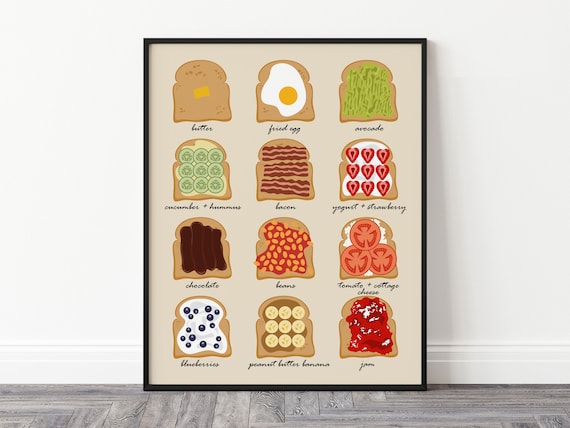The image depicts a framed art piece featuring twelve illustrated slices of toast, each uniquely topped and labeled in black cursive script. The poster is rectangular, encased in a thin black frame, and has a beige background. The frame leans against a white wall on a gray wooden-tiled floor. Each row of toast aligns in a grid with three columns and four rows, showcasing a variety of colorful toppings. The slices from left to right and top to bottom are adorned as follows: 

1. A piece with a pad of butter labeled "butter."
2. A slice with a poached egg labeled "poached egg."
3. A slice with avocado labeled "avocado."
4. A slice with cucumber and hummus labeled "cucumber and hummus."
5. A slice with bacon labeled "bacon."
6. A slice with yogurt and strawberry labeled "yogurt and strawberry."
7. A slice with chocolate labeled "chocolate."
8. A slice with beans labeled "beans."
9. A slice with tomato and cottage cheese labeled "tomato and cottage cheese."
10. A slice with a white cream and blueberries labeled "blueberries."
11. A slice with peanut butter and banana labeled "peanut butter and banana."
12. A slice with jam labeled "jam."

The art piece incorporates a mix of red, orange, yellow, green, dark purple, brown, beige, black, and gray colors, making it a fitting and decorative addition to a kitchen setting.